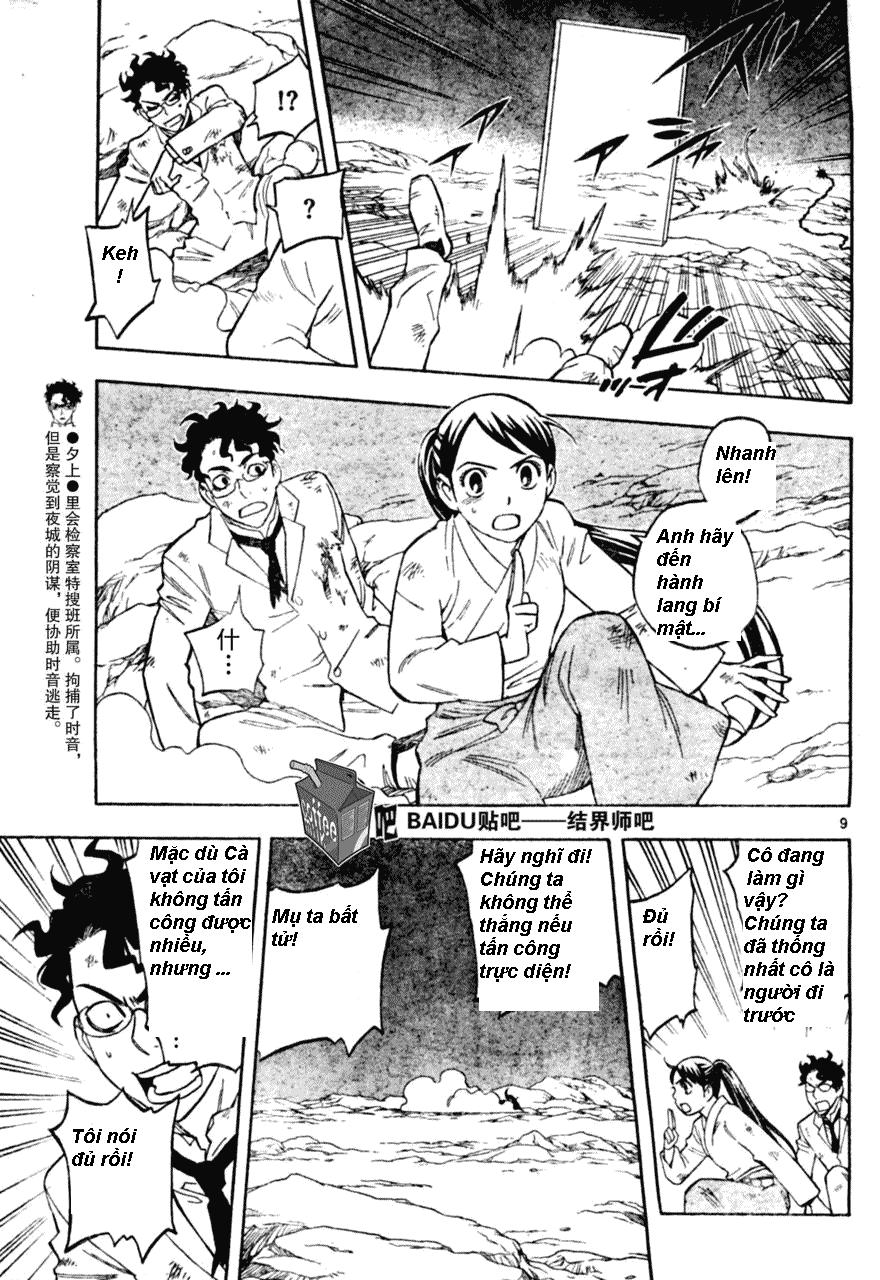The image is a black-and-white comic strip featuring six panels with a serious tone. The characters appear to be drawn in an anime style, with exaggerated eyes, and the text is in Vietnamese, overlaid onto what seems to have originally been Japanese. 

In the first panel, a disheveled man with black scraggly hair is lying down in a rocky area, looking dirty and as though he has been caught in a windy, harsh environment. His arm is raised defensively. The background suggests a stormy day.

The second panel depicts an explosion, with debris, including a rectangular object, flying through the air. The man’s feet are also visible, showing he's been thrown by the blast.

In the third panel, the man is sitting on the ground, looking worn out, and a woman appears beside him. Her clothes are tattered, and she has her mouth open, saying something in Vietnamese.

The fourth panel is a close-up of the man, who seems to be speaking, his expression determined despite his exhausted appearance.

The fifth panel shows a desolate landscape with no characters present but includes speech bubbles with Vietnamese text, suggesting the conversation continues off-screen.

In the sixth and final panel, the woman, with her index finger raised, seems to be making a point or giving instruction, while the man stands behind her.

Throughout the comic, there's an integration of the word "Baidu," a recognizable search engine brand, and Asian fonts, hinting at a mix of cultural elements.